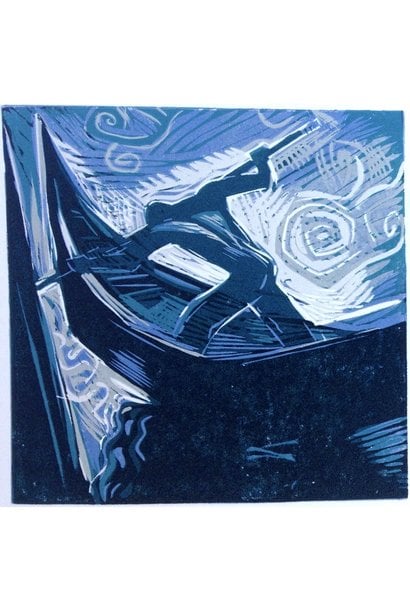This is a highly stylized, almost comic book-like painting of a man in a small, single-person canoe. The scene suggests a stormy night at sea, with a predominantly dark, moody palette of blacks, dark blues, and whites, while lighter blues add depth and detail. The background is filled with swirling white and light blue patterns, evocative of strong winds and turbulent waters, which heighten the sense of motion and urgency.

In the center of the painting is the man, illustrated in silhouette with dark blue shading that reveals the straining muscles on his bare torso. He is holding a pole or oar over his shoulders, leaning forward, and pushing against a larger surface, possibly rocks, as if trying to navigate through or escape the tumultuous environment. The canoe itself is mostly black, with hints of blue detailing and a pointed, high front, cutting through the depicted waves. Lines emanate from the boat's bow, suggesting it's making progress through the rough sea. The entire composition is dynamic, conveying movement and the raw force of nature.